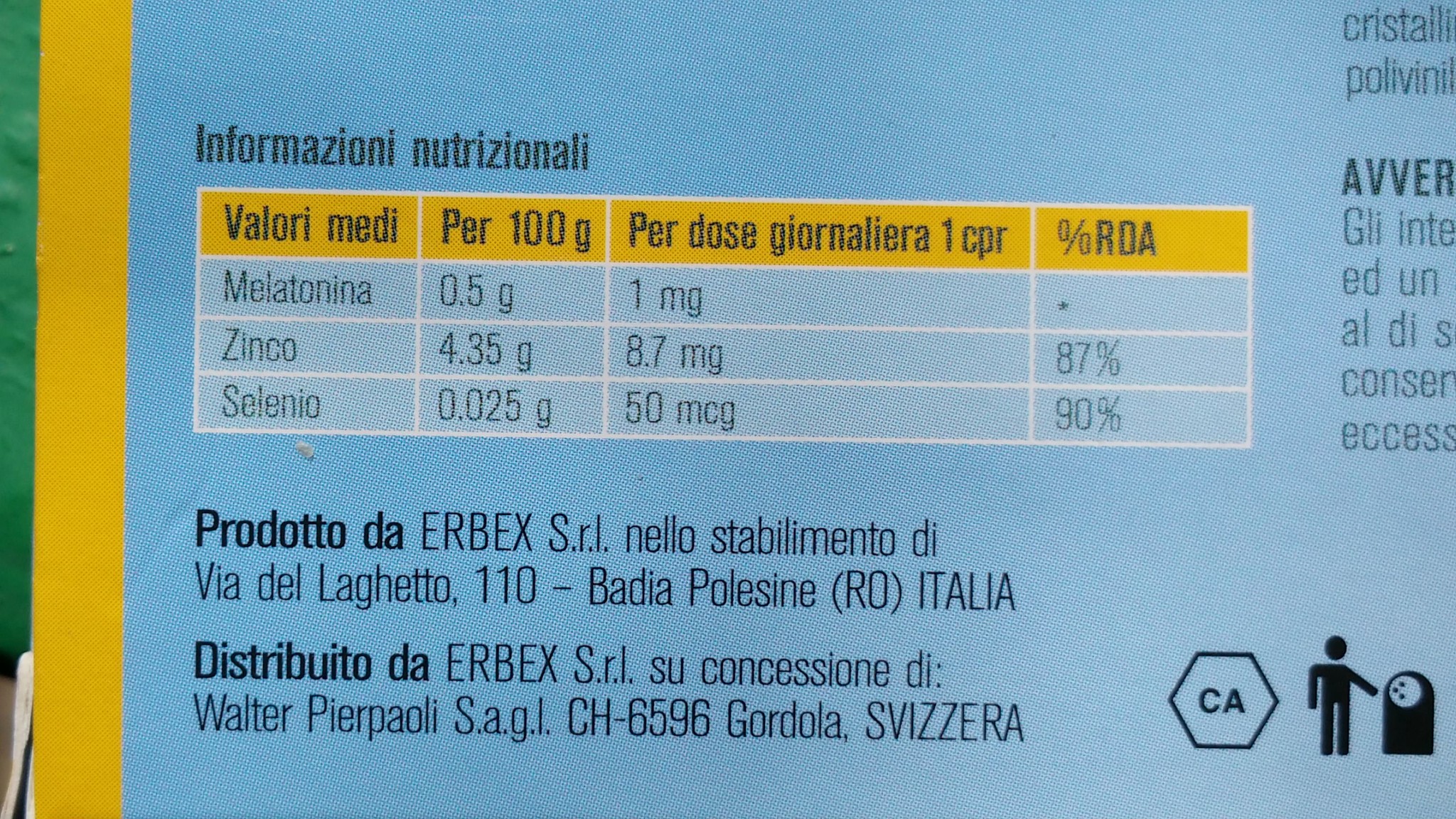This image displays the nutritional information on the back of a blue and yellow package, likely of Italian origin, as indicated by the Italian text. The packaging features a green trim and a thicker white trim at the edge. Prominently, it states "Informazione Nutrizionale" (Nutritional Information) and includes details presented in a structured table format. The table highlights nutritional values per 100 grams and per daily dose, with measurements for ingredients such as Melatonina (Melatonin), Zinco (Zinc), and Selenio (Selenium). Specific values listed include Melatonina at 0.5 grams per 100 grams and 1 milligram per dose, Zinco at 4.35 grams per 100 grams and 8.7 milligrams per dose, and Selenio at 0.025 grams per 100 grams and 50 milligrams per dose. The percentages of the Recommended Daily Allowance (RDA) are also provided, with Melatonina marked by an asterisk, Zinco at 87%, and Selenio at 90%. 

Additionally, the packaging includes manufacturing details, indicating it is produced in Badia Polesine, Italy by Urbex and distributed from Gordola, Switzerland. A hexagonal symbol with "CA" is present, along with an icon of a person disposing of waste in a trash can, signifying proper disposal instructions.